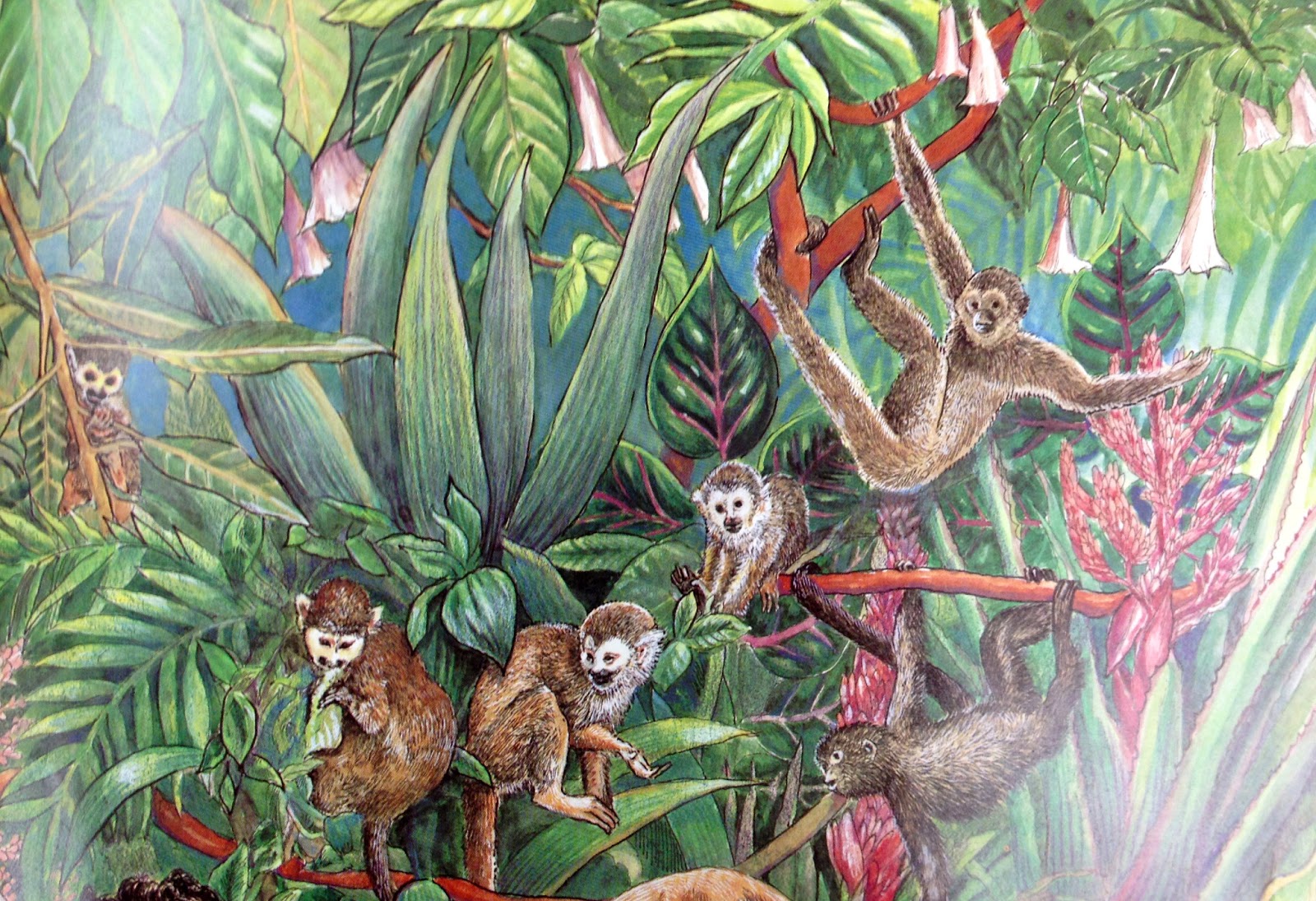The image is a detailed, cartoon-like painting of a vibrant jungle scene teeming with wildlife. At the center of the composition are several playful and active brown monkeys, each exhibiting distinctive facial markings. On the left side, four monkeys have white patches around their eyes, contrasting with their brown fur, while on the right, two other monkeys feature a more tan coloration around their eyes. The jungle itself is lush with enormous green leaves projecting outward, some appearing larger than life in comparison to the monkeys. The foliage includes various types of vegetation, with long green leaves and massive green blades scattered throughout. Adding to the scenic beauty are light pink, trumpet-shaped flowers and white bell-like flowers hanging from the upper part of the painting. The monkeys are shown interacting with their environment, some swinging from tree branches with their tails wrapped around them, creating a lively and dynamic atmosphere.